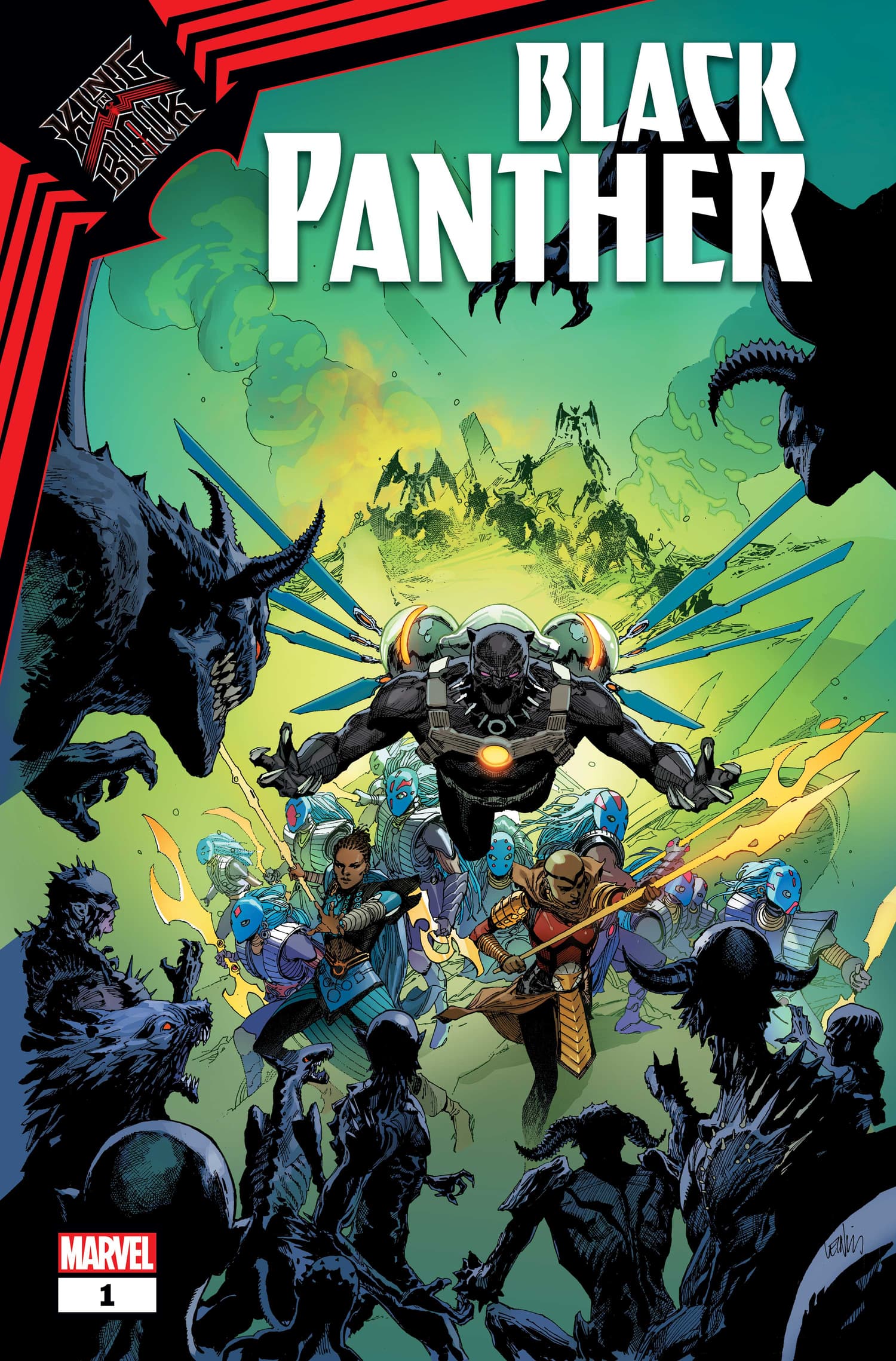The image is the cover of a comic book, featuring vibrant and chaotic artwork. At the top right, the title "BLACK PANTHER" is written in large, white block letters, right-aligned across two lines. In the top left corner, a black shape outlined in white contains the words "KING BLACK" in bold, black letters. Striking red lines emanate from either side of the black shape, creating an upside-down V shape. Below the title, the central image showcases Black Panther, who appears to be flying towards the viewer with arms outstretched, emanating blue lines from a jetpack-like device on his back. He is adorned with gray straps around his shoulders and chest, and a glowing yellow circle in the center of his chest. Surrounding him are numerous characters, including a woman in blue wielding a spear and another bald woman dressed in red and gold, also holding a spear. At the bottom of the cover, the foreground features a horde of monstrous creatures, some with horns and others resembling skinny werewolves, poised to attack. In the lower left corner, a small red rectangle bears the white MARVEL logo, with a white horizontal rectangle beneath it containing a black number "1." The overall scene is one of intense action and vivid colors, encapsulating the dynamic essence of the comic book genre.